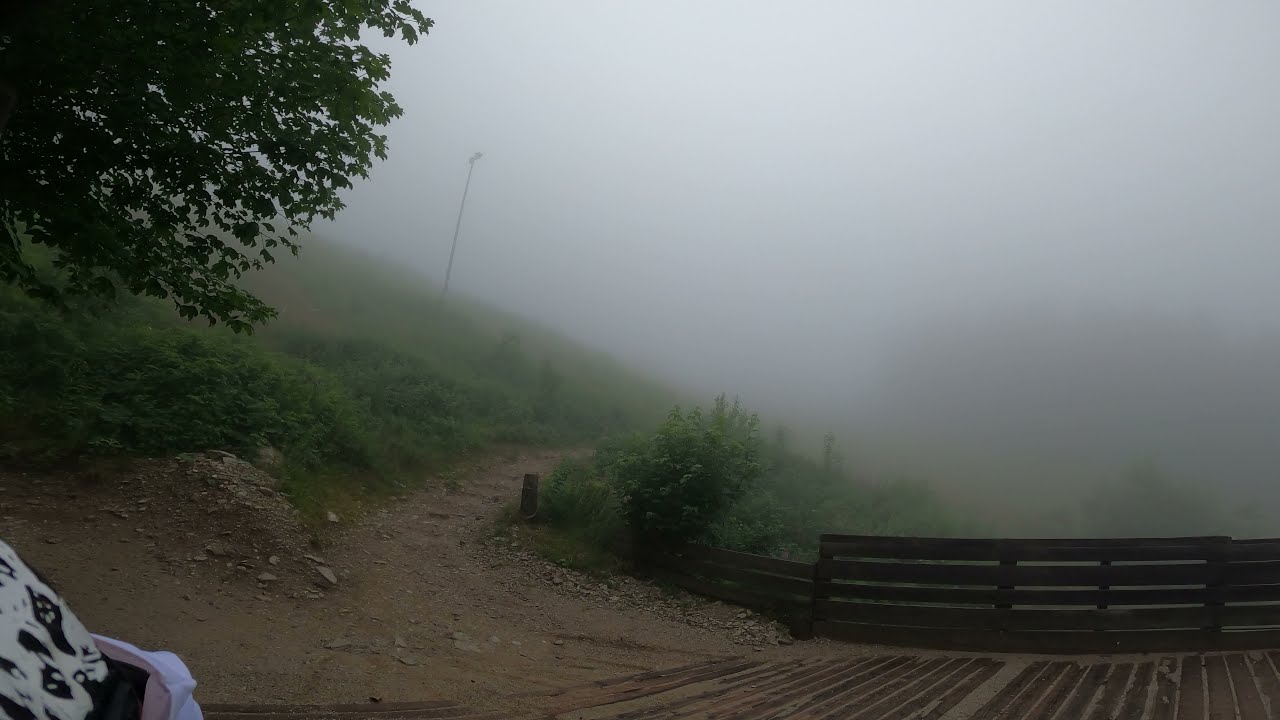A thick fog blankets the scene in this outdoor daytime photograph, making visibility extremely limited and creating a gray, misty atmosphere. A grassy hill dominates the lower portion of the image, transitioning into a brown dirt area with a gravel footpath running diagonally through it. To the right, a dark wooden fence borders what appears to be a small pedestrian bridge with parallel slats, possibly wooden or metal. In the background, a tall pole, likely a telephone or light pole, stands obscured by the dense fog. A solitary tree rises from the left, its upper branches fading into the mist. The bottom left corner reveals a hint of a person's light pink clothing and possibly a white-sleeved garment with black patterns, adding a subtle human element to the tranquil, foggy landscape.